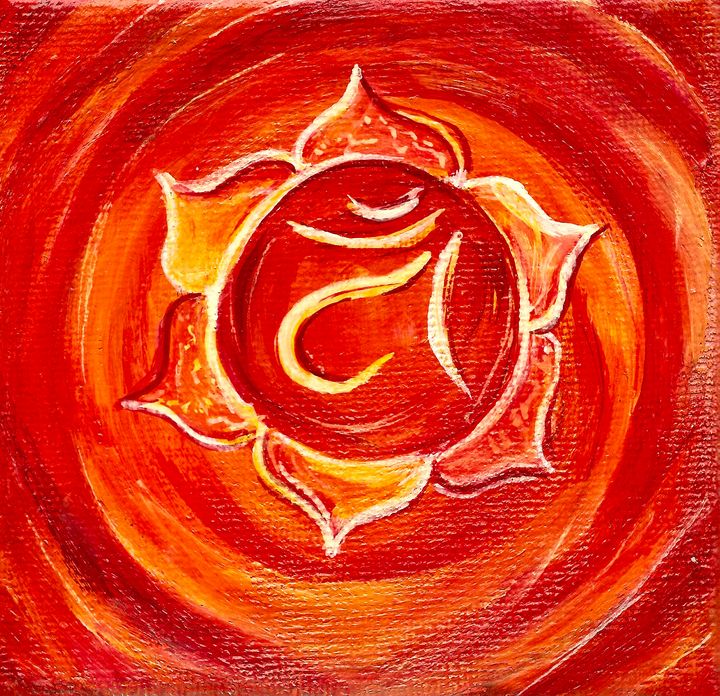The image appears to be a detailed drawing or painting predominantly in shades of red, orange, and yellow with intricate swirls and patterns. The central element features a large red circle with a white outline, resembling a stylized flower. Inside the circle, numerous white and yellow swirling lines create dynamic shapes, including a hook-like curve and additional delicate spirals. Surrounding the central circle are six petal-like extensions, each filled with a blend of red, orange, and yellow hues, and also outlined in white. The overall composition of the artwork seems reminiscent of a vibrant sun or a blossoming flower, set against a background of bold, circular red strokes. The entire design is enclosed within a square frame, giving it a cohesive and framed appearance. The image does not contain any text or additional objects, and the colors outside the main palette are sparse, emphasizing the dominance of red tones and the intricate detailing within the central floral motif.